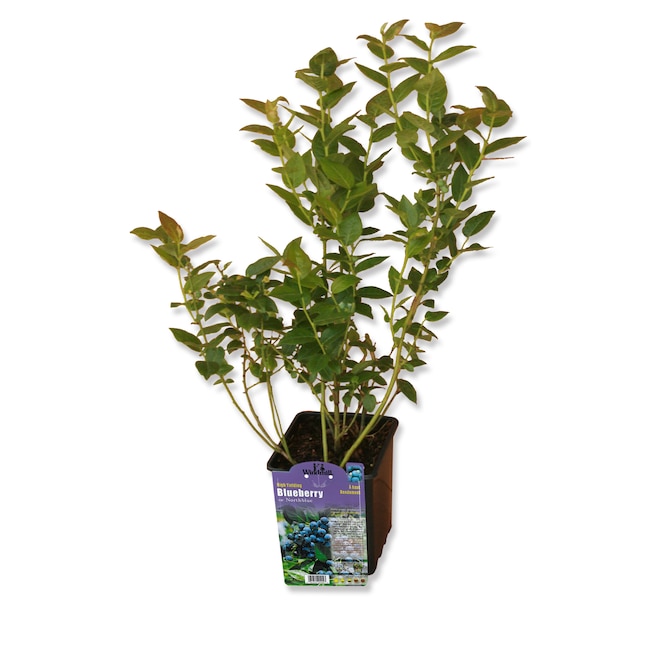The photograph captures a young, vibrant blueberry plant against a seamless white background, making it appear borderless on the computer screen. The plant is neatly housed in a small, approximately four-inch black nursery container typical of garden centers—those familiar, low-cost, recyclable plastic pots. Attached to the front of this pot is a branded, plastic tag displaying an image of blueberry fruits and the plant's name, complete with a UPC code and likely planting instructions on the reverse side. The healthy, multi-stemmed plant stands distinguishably with about 2-3 main stems and 6-7 branching stems that range in height from shorter ones at the front to nearly double in length at the back. The lush leaves exhibit a fresh, green texture, with the tips of the newest growth tinged a delicate red, suggesting robust health and vitality. Though no berries are present yet, the image on the tag hints at the promise of future fruit, making this young plant ready to be taken home and planted in a garden.